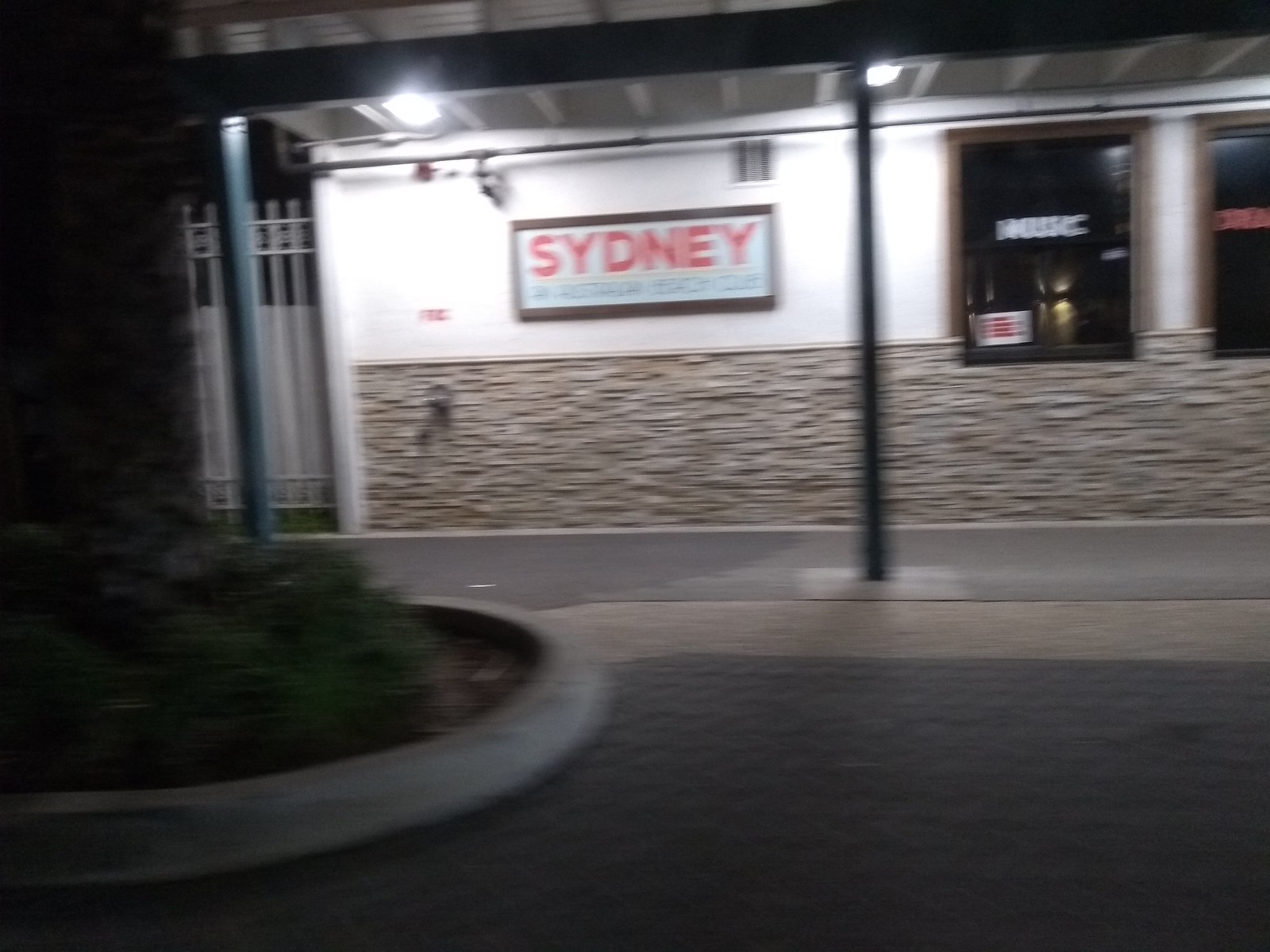This nighttime photograph captures the front façade of a small building with a prominent red sign that reads "Sydney." Below the main sign, there's smaller text that is not clearly legible in the image. The building is likely located in Australia. To the right of the entrance, there are windows with dark interiors; one of these windows has white lettering that spells out "Music." The illuminated exterior of the building stands out against the darkness. A walkway bordered by a curb runs along the front of the building, and on the left side of the photo, there are bushes and a tree adding a touch of greenery to the scene.